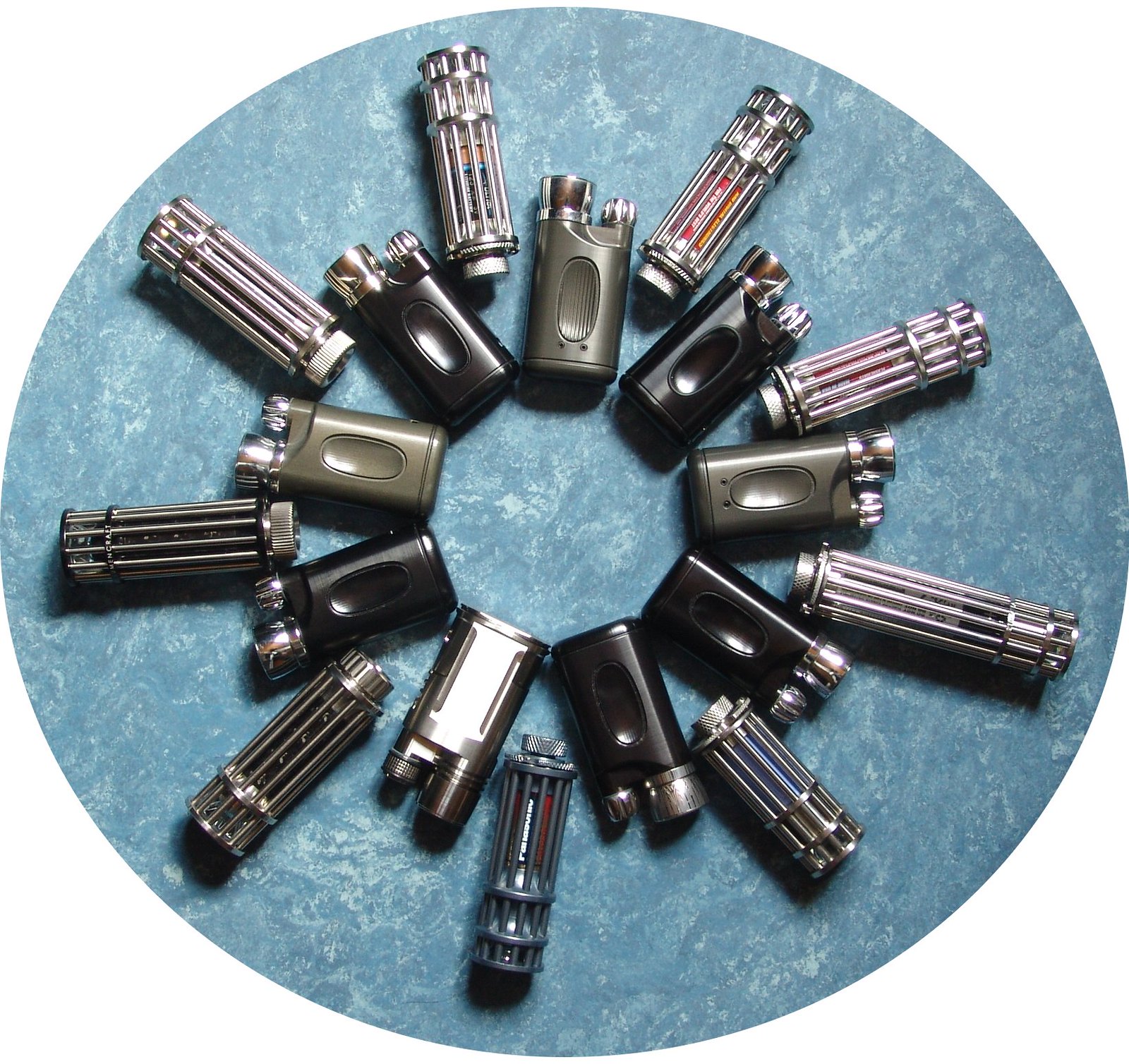The image displays an intricate arrangement of various devices, likely lighters, meticulously positioned in a circular pattern atop a blue, marble-textured table. The core of the design features smaller, black and olive green lighters with a vertical, ovular circle down their middles. Surrounding this core, a series of cylindrical devices, resembling mechanical components with visible AA batteries encased in metal rods, extend outward, positioned like the hands of a clock at the 11, 1, 2, 4, 5, 6, 8, 9, and 10 positions. The image's composition combines the rotational design with a dynamic interplay of green, black, and one striking silver device, creating a visually captivating starburst effect.